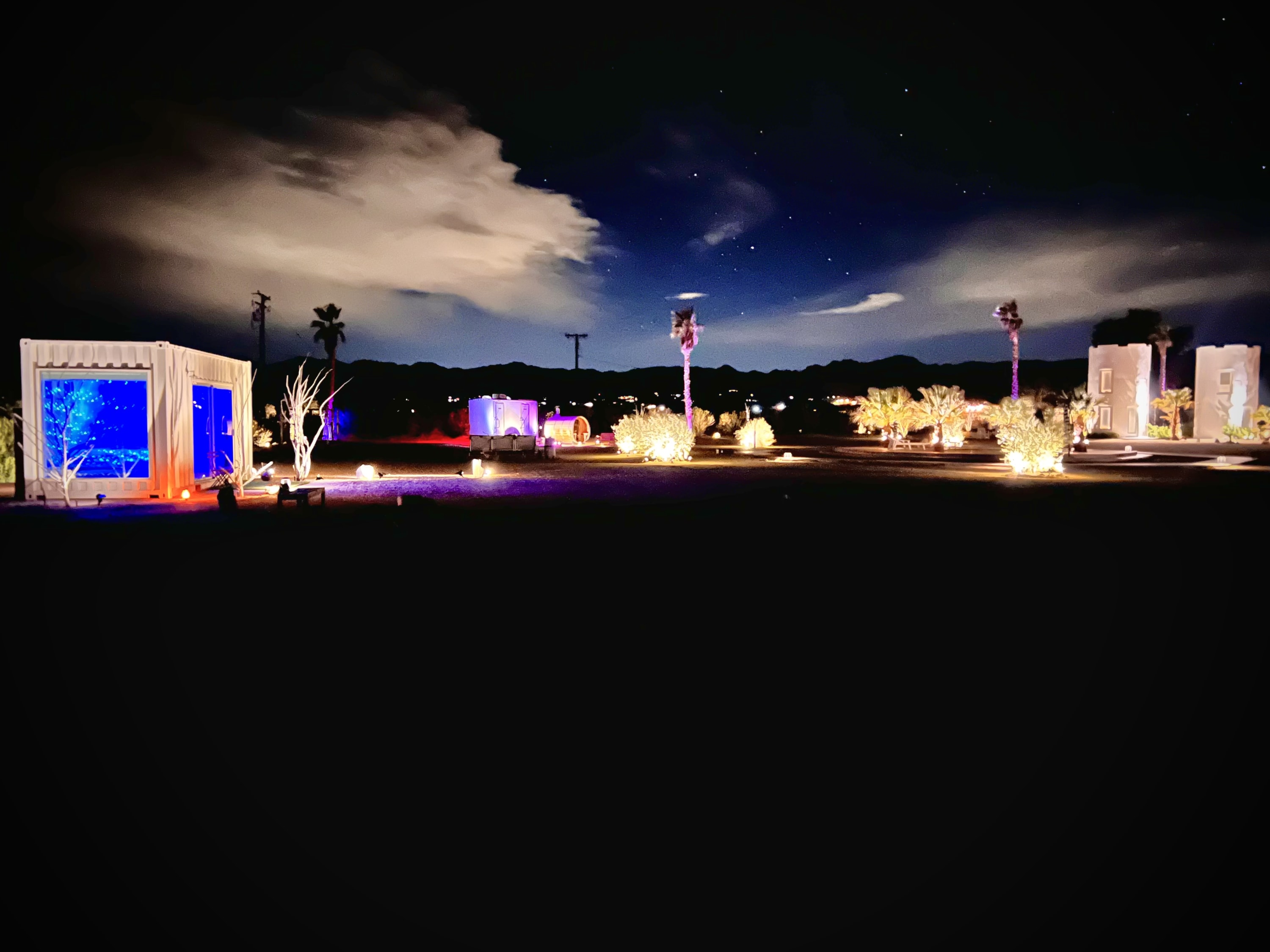The image captures a nighttime scene in a desert-like environment, devoid of light pollution, showcasing a richly lit setup for what seems to be a party or event. The sky is dark, dotted with stars and clouds. In the foreground, the area is almost entirely black, punctuated by sconce lighting that highlights sections of the ground and structures. 

Prominent are several small buildings adorned with vibrant, colorful lights such as blue, pink, red, purple, and yellow. One building features blue walls, illuminated by these lights, standing near dead trees that blend naturally into the lit environment. There are also palm trees with their bases surrounded by glowing bushes, and their leaves lit up in various colors.

The scene extends to what appears to be a parking lot with two white walls surrounded by glowing white bushes. In the far background, there are hints of a mountainous or hilly region with scattered lights, suggesting distant population centers. Overall, the image resembles a festive setup, possibly akin to a large music festival like Coachella, set against a dynamic and colorful desert nightscape.